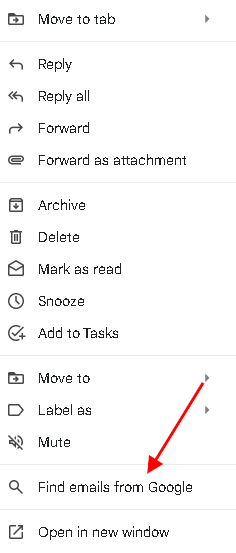Screenshot of an Email Menu Interface

The screenshot captures an email menu interface, possibly from Yahoo Mail, presented on a white background with black text. The menu options are as follows, listed top to bottom:

1. **Move to tab**: Accompanied by an arrow pointing to the right.
2. **Reply**: Marked with a reverse arrow.
3. **Reply All**: Indicated by a double reverse arrow.
4. **Forward**: Represented by an arrow pointing right.
5. **Forward as attachment**: Depicted with a paperclip icon.
6. **Archive**: Illustrated by a box pointing downwards.
7. **Delete**: Shown with a trash can icon.
8. **Mark as read**: Displayed with an open mail envelope.
9. **Snooze**: Depicted with a clock icon.
10. **Add to tasks**: Represented by a circle with a check mark.
11. **Move to**: Accompanied by a file icon with a move arrow.
12. **Label as**: Shown as a blank squared triangle.
13. **Mute**: Indicated with a speaker having a cross-out symbol.

Additionally, the menu contains:

- **Find emails from Google**: Marked by an hourglass icon.
- **Open in new window**: Located at the bottom of the list.

A red arrow is pointing from the "Move to" option down to "Menu," highlighting the "Find emails from Google" option with an hourglass icon and "Open in new window."